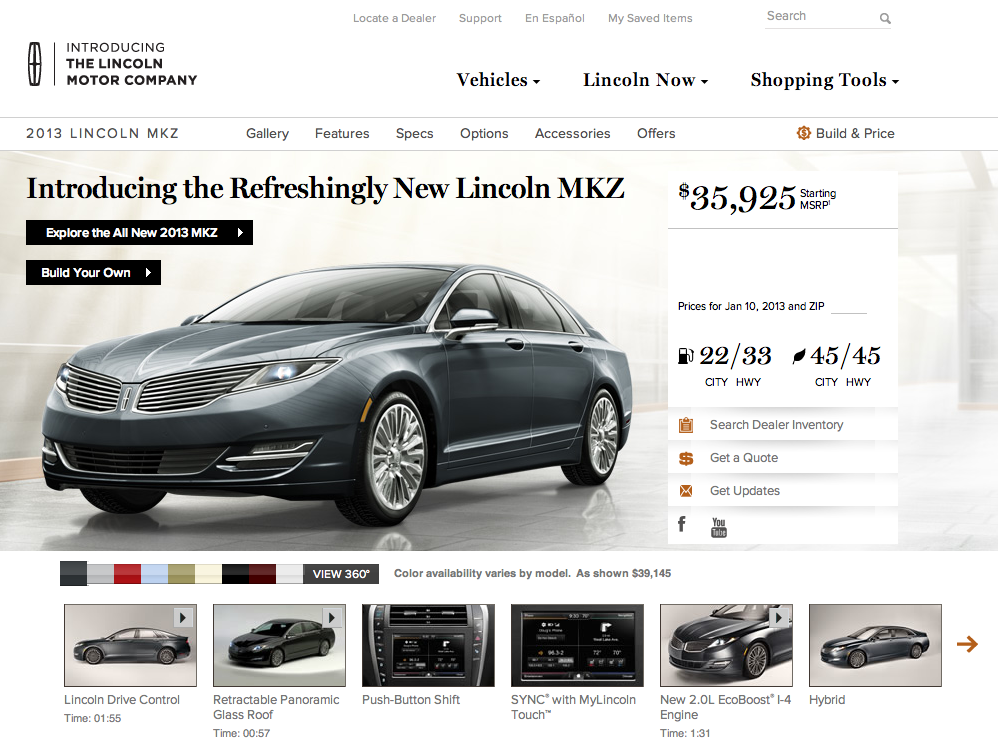This advertisement by Lincoln introduces the Lincoln Motor Company and showcases the all-new 2013 Lincoln MKZ. The promotional text highlights features, specifications, options, accessories, and special offers for the vehicle. Viewers are encouraged to explore the MKZ's gallery, build and price their own model, and utilize various shopping tools available.

The image prominently displays a slate blue 2013 Lincoln MKZ, emphasizing its sleek and modern design. Key details include city mileage rated at 22 miles per gallon, and highway mileage rated at 33 miles per gallon, with equivalent measurements in kilometers also provided. The advertisement encourages potential buyers to search dealer inventories, get quotes, receive updates, or visit further media on YouTube.

The MKZ is presented in an array of colors, including blue, gray, red, baby blue, taupe, cream, navy blue, and dark brown. It comes equipped with advanced features like Lincoln Drive Control, a retractable panoramic glass roof, push-button shift, and the MyLincoln Touch system. The vehicle boasts a new 2.0 EcoBoost 1.4 engine and is also available as a hybrid model.